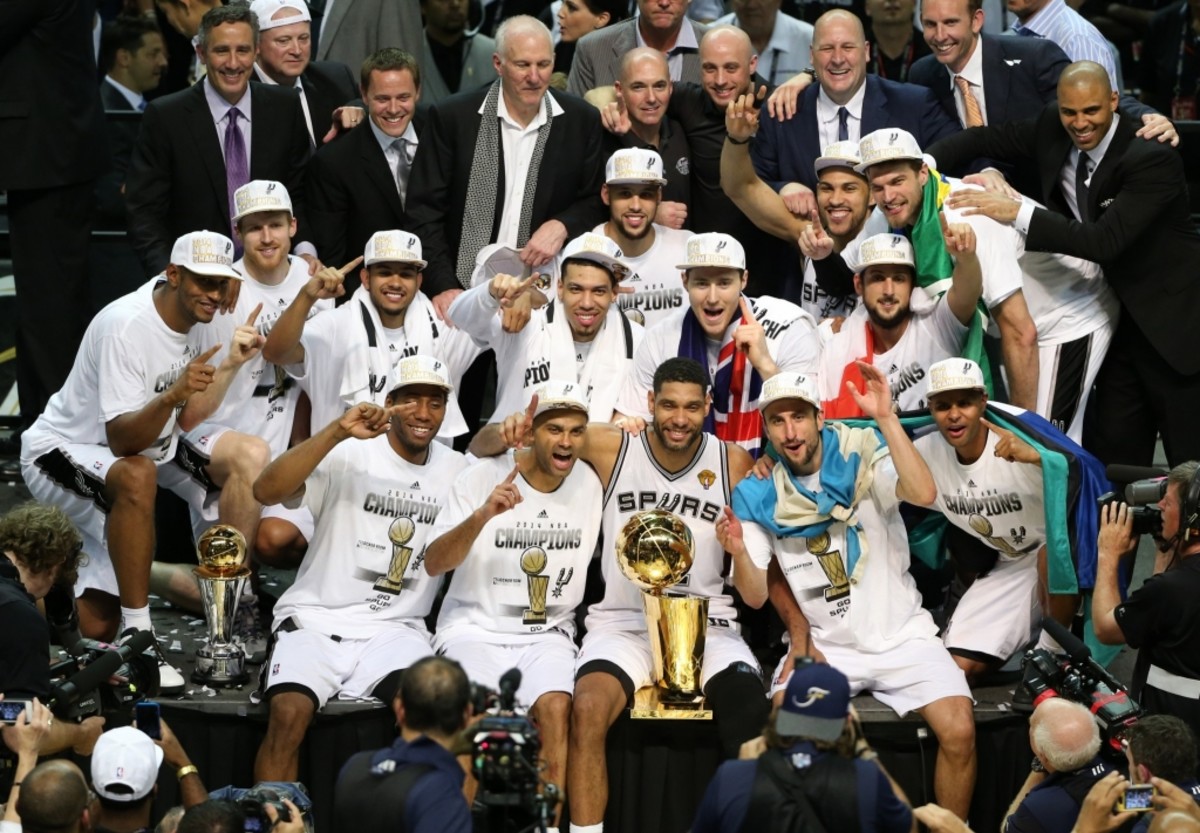The image showcases the victorious San Antonio Spurs basketball team celebrating their NBA Finals win. The entire team is posing, each player wearing white clothing—some in sleeveless jerseys with "Spurs" emblazoned on the front, and others in short-sleeved shirts that highlight "NBA Champions" along with a championship trophy graphic. The players have their index fingers raised, signifying their number one status. Centrally placed, in the front row, are two gleaming golden trophies—one held by a player in the center and another nearby on the left. Surrounding the team are numerous journalists capturing the moment, while in the background, the coaching staff and possibly team owners are dressed in formal black suits with ties, adding a formal touch to the celebratory scene. The vibrant setting, filled with colors like white, black, purple, red, light blue, and green, appears to be courtside, immediately following their triumphant game. The atmosphere is bustling and charged with excitement, with little empty space, emphasizing the crowded and jubilant environment.